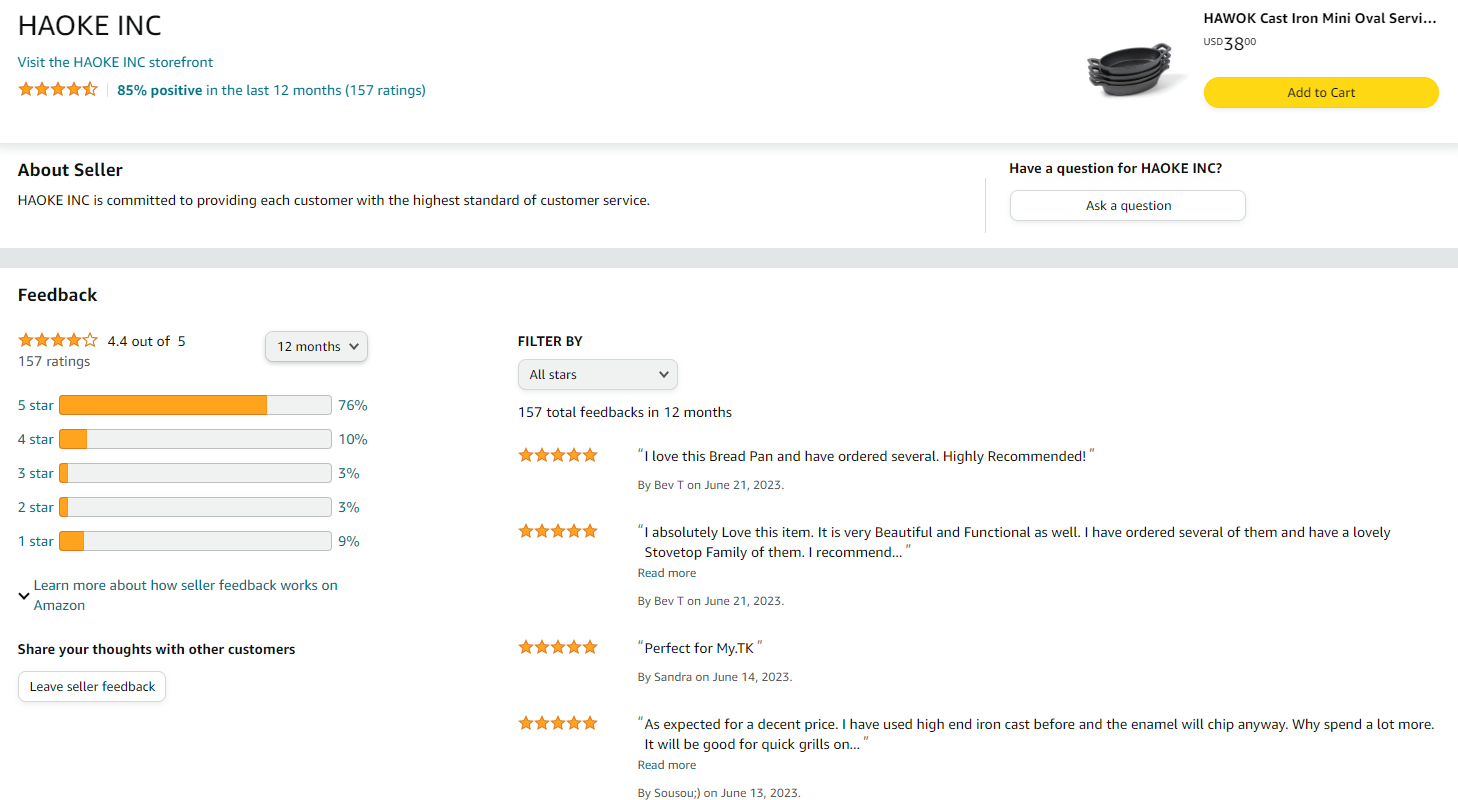**Detailed Caption for Amazon Product Feedback Screenshot:**

The screenshot depicts a product feedback page on Amazon, focusing on the "Hawwok Cast Iron Mini Oval Service," priced at USD 38. A small image of the product is visible in the top right corner, showing a black cast iron kitchen set. To the right of the image, there is an "Add to Cart" button. The seller's information is listed on the left-hand side, starting with "Hay Oak Inc.," with a link to visit their storefront. 

The product has an overall star rating of four and a half stars based on 157 ratings, with 85% positive feedback in the past 12 months. Beneath the seller information, there's an "About Seller" section stating, "Hay Oak Inc. is committed to providing each customer with the highest standard of customer service." There is also a "Have a question for Hay Oak Inc.? Ask a question" prompt.

The feedback section shows an average rating of 4.4 out of 5 stars from 157 ratings over the last 12 months. A dropdown menu allows users to adjust the time frame of the feedback being viewed, defaulting to 12 months. Star ratings are broken down with percentages for each category: 5 stars, 4 stars, 3 stars, 2 stars, and 1 star. There is also a "Learn more about seller feedback" link explaining how feedback works on Amazon and encouraging users to share their thoughts with other customers.

A box is available for leaving seller feedback. To the right, there's an option to filter feedback by star rating, with a dropdown menu currently set to "All Stars." The total feedback count of 157 within the last 12 months is prominently displayed.